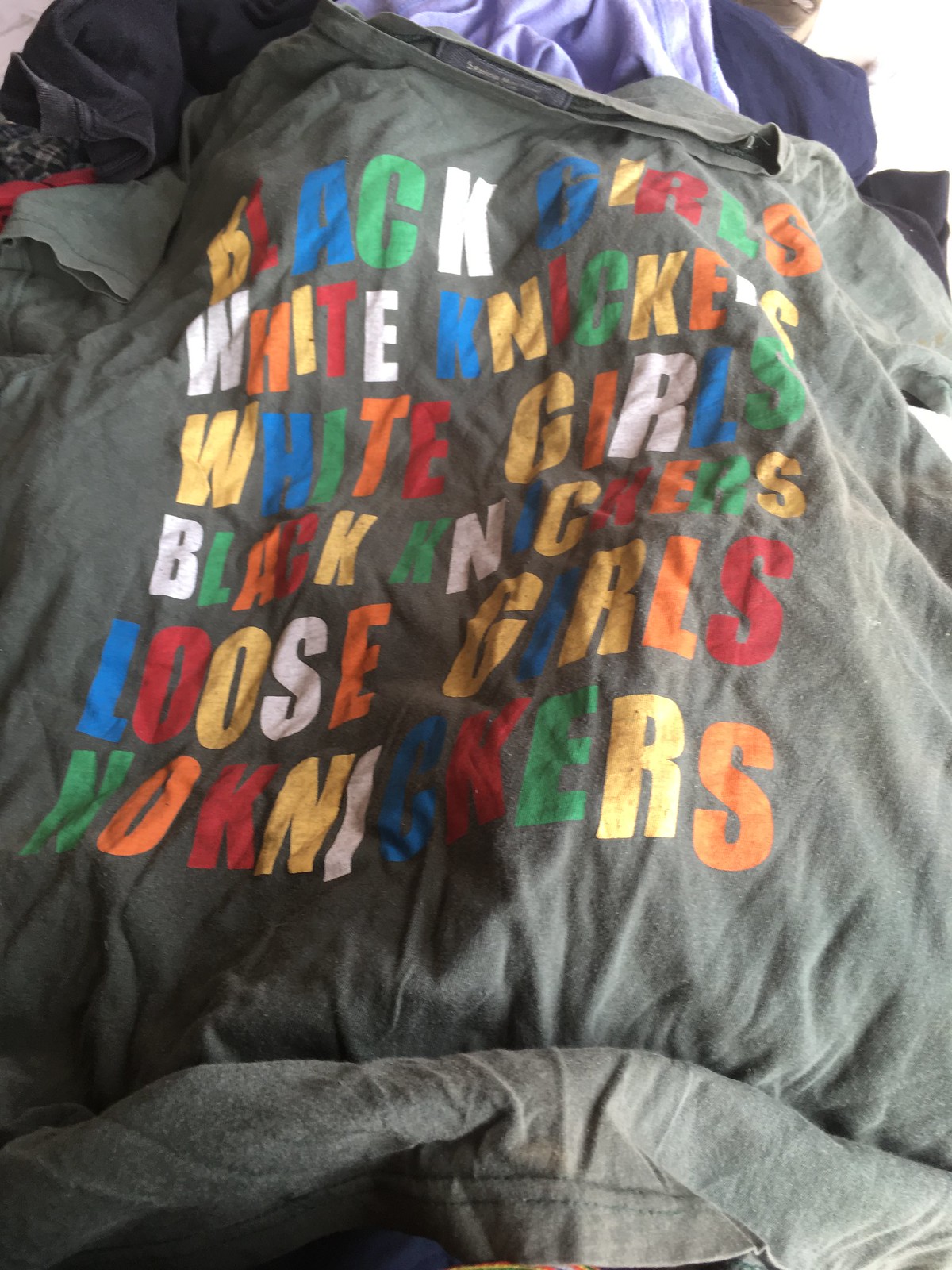The image depicts a wrinkled gray shirt lying on a disorganized pile of clothes. The shirt features a multicolored text on the front, with hues of white, yellow, red, blue, and green, though the exact phrasing is unclear. Words such as "black girls" and "white girls" are partially readable, alongside other text that is somewhat distorted and hard to make out. In the background, a purple shirt, blue shorts, and part of a white wall are visible at the top right corner of the image.